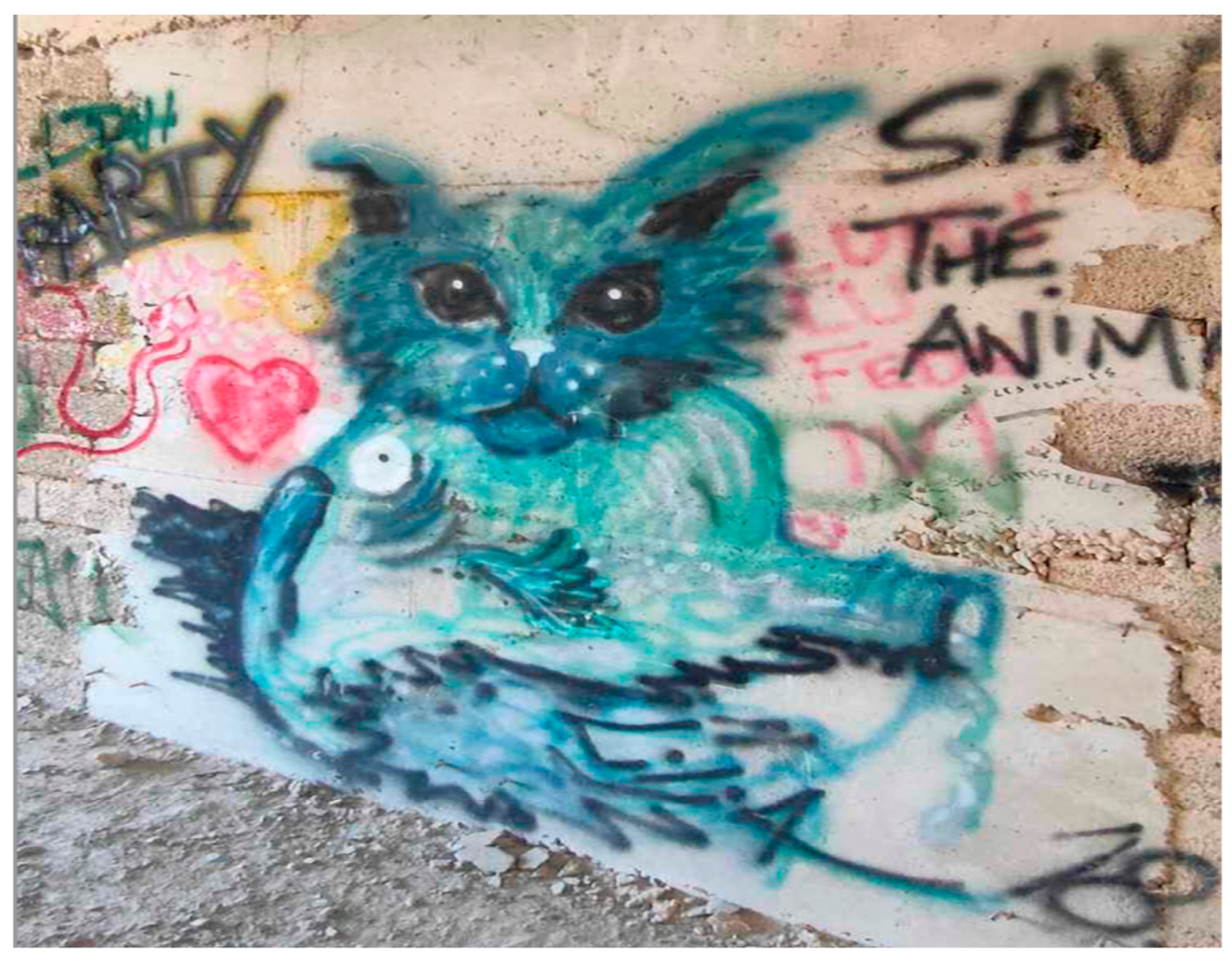The image depicts a mural on an old, crumbly brick wall smeared together to create a flat surface under layers of paint. The central focus is a large blue cat with black eyes facing the camera, exuding a sad expression. Surrounding the cat, the wall is adorned with various graffiti elements. To the right of the cat, the partially visible text "save the anim" is written in black spray paint, suggesting an animal conservation message. To the left is a prominently painted red heart with a yellow outline and the word "party" in black. Additional graffiti includes red and blue squiggles, a pink heart, and a green "OK". The wall shows signs of wear with crumbling edges, and the ground in front consists of dirt or clay. In the bottom corner of the mural, the number "18" is inscribed without clear context. The mural is painted on a light gray brick wall, weathered and infused with artistic expressions.